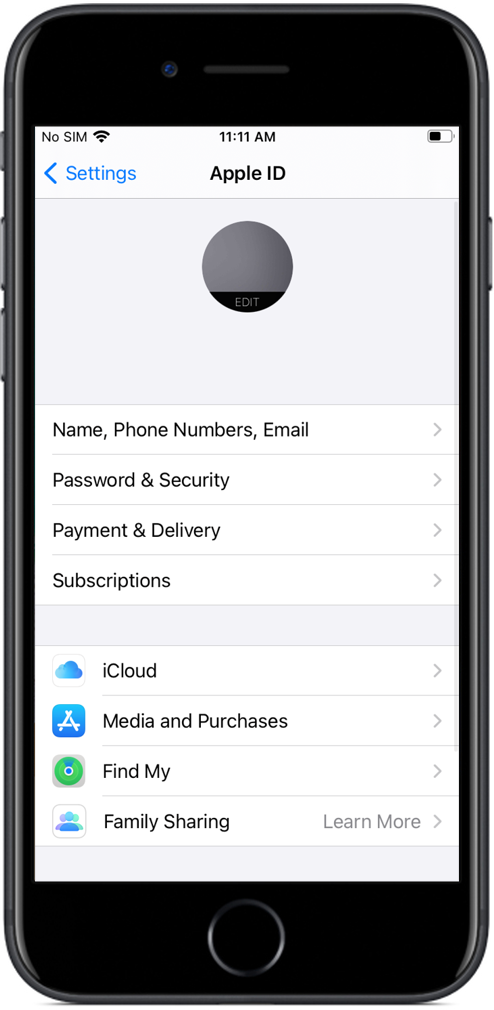This screenshot from a cell phone depicts the Apple ID login screen. The device's status bar shows 11:11 AM, a half-full battery, and no SIM card installed. At the top of the login interface, "Apple ID" is written, accompanied by a blank, gray circular avatar placeholder and a blue settings button to its left. Below this, the user is prompted to enter their name, phone number, and email, followed by their password.

The middle section offers various options, including "Payment & Delivery" and "Subscriptions." Following this, we see the "iCloud" section with a cloud icon, "Media & Purchases" marked by a blue icon with white text, and "Find My" displaying a green icon and black text. Beneath these, "Family Sharing" is noted with a blue icon and a lighter black text that reads "Learn More."

This comprehensive view captures the attempt to log into an Apple ID on a phone without a SIM card, potentially hindering the process. The screen, replete with typical iOS interface elements, details all necessary login fields and additional account management options.